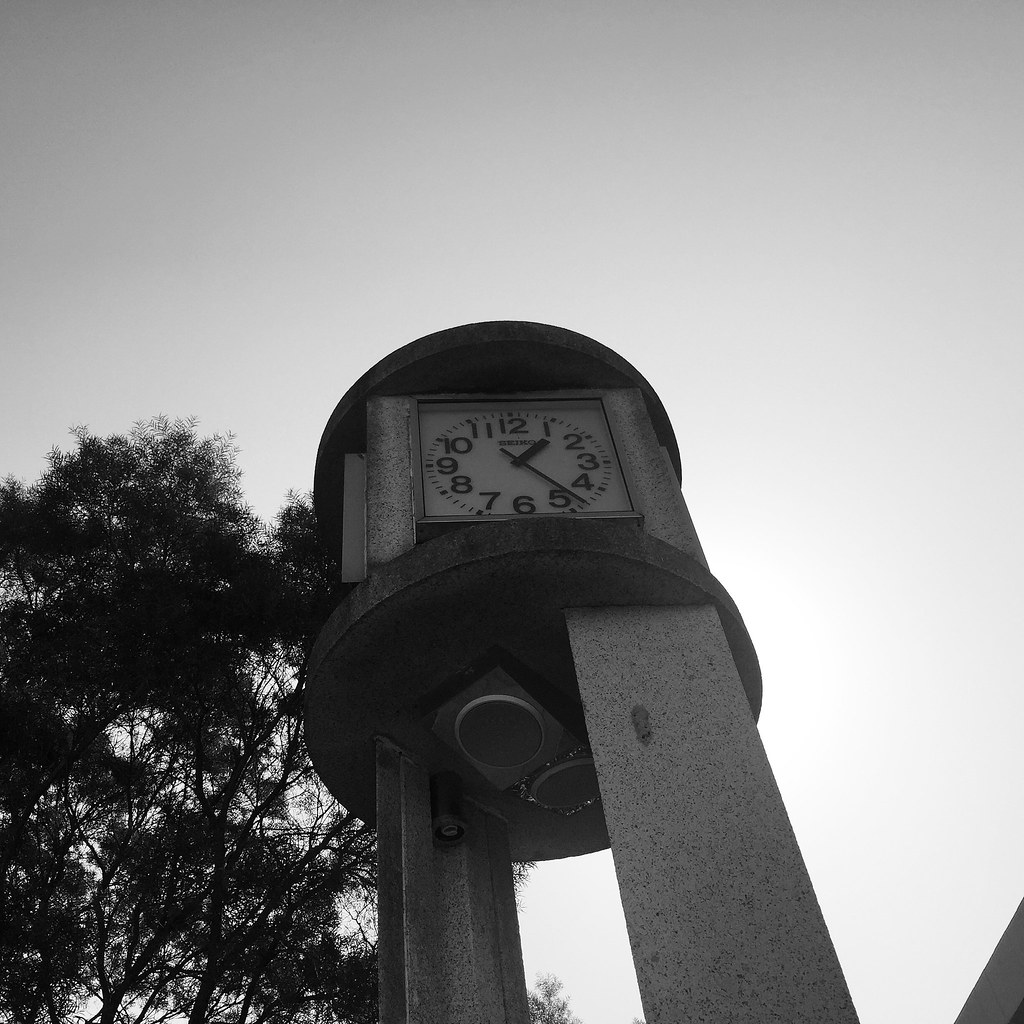This black-and-white photograph captures a striking clock tower from a low-angle perspective, emphasizing its towering presence against the sky. The structure, which is reminiscent of a traditional clock tower, appears to be constructed from robust concrete or metal posts that support a thick disc around which the clock face is centered. Adjacent to the clock tower and slightly behind it to the left stands a tall tree, providing a sense of scale and highlighting the tower's impressive height.

The clock face itself is square and numbered from 1 to 12, with small dashes indicating the minutes and hours on the outer ring. The time displayed is 1:25, with the clock hands clearly visible against the monochrome backdrop. At the top center of the clock face is a logo, though it is unreadable in the photograph.

The overall lighting and shadows suggest that the photo was taken during the daytime, perhaps in the late afternoon or early evening, as the light is somewhat dim, hinting at the onset of dusk. The stark contrasts and architectural details are beautifully accentuated by the black-and-white format, giving the image a timeless and evocative quality.